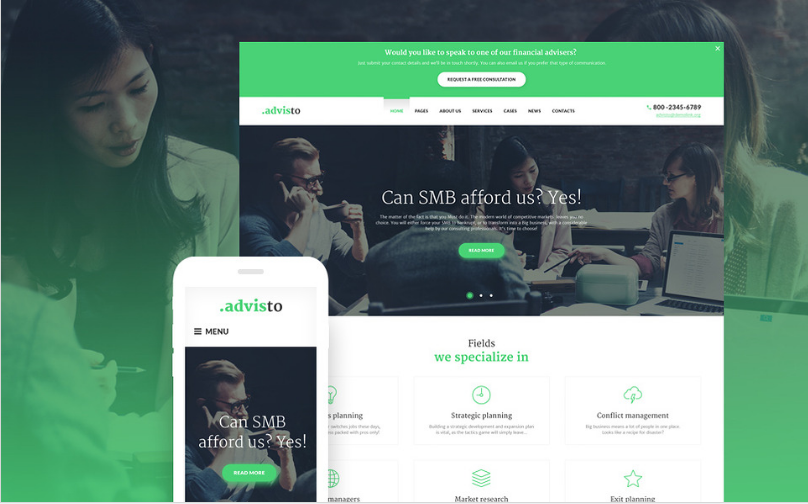The image depicts a website titled "Advisto." The "advis" portion of the name is highlighted in green, while the "to" is in black. At the top of the page, there is a prompt that reads, "Would you like to speak to one of our financial advisors?" Due to the low-resolution quality of the image, some of the text is difficult to discern. Under this prompt, there is a white button labeled "Request a free consultation." 

The site features multiple navigation tabs within a white area, including "Home," "Pages," "About Us," "Services," "Careers" or possibly "Cases" (the text is hard to make out), "News," and "Contacts." A phone number, 800-2345-6789, is also listed. Below this information, there is an image showing a group of people engaged in some form of work activity.

A section of the website poses the question, "Can SMB afford us?" with the affirmative answer "Yes." This section includes a white paragraph of text and a green "Read More" button. Additionally, there is a list of fields in which the company specializes, such as strategic planning, conflict management, market research, exit planning, and several more. Each field is accompanied by a small icon for visual representation.

The website is also shown in a mobile phone interface, maintaining the same essential content: the prompt "Can SMB afford us? Yes" and the "Read More" button. The overall layout suggests a comprehensive, albeit visually outdated, financial advisory service platform.